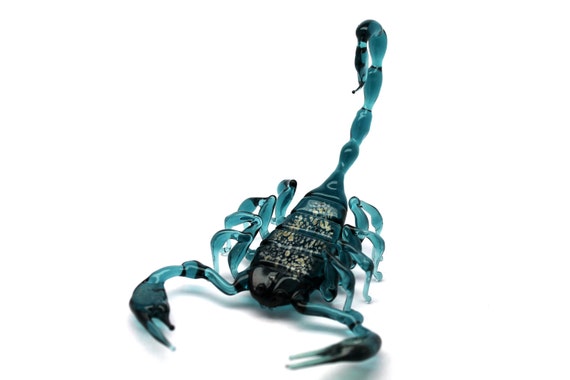The image depicts a detailed art piece of a scorpion that is not real but crafted from either resin or glass. This stunning representation features a primarily teal or turquoise hue mixed with darker tones along its body and pinchers. The central body area showcases hints of gold, adding a glittery accent which contrasts beautifully with the dark and vibrant teal shades throughout. The scorpion's tail, curving high above as if ready to strike, and its poised pinchers are noticeably darker, emphasizing a striking look. Beneath its folded legs, which are meticulously arranged on both sides, a shadow is cast on the completely white background, indicating light coming from above. The scorpion, with its sharp tail tip and lifelike stance, faces the camera, capturing a sense of vivid realism despite being a man-made creation. This piece, detailed in turquoise, black, and gold, exudes an artistic flair, making it appear almost as a product to be showcased in an advertisement.